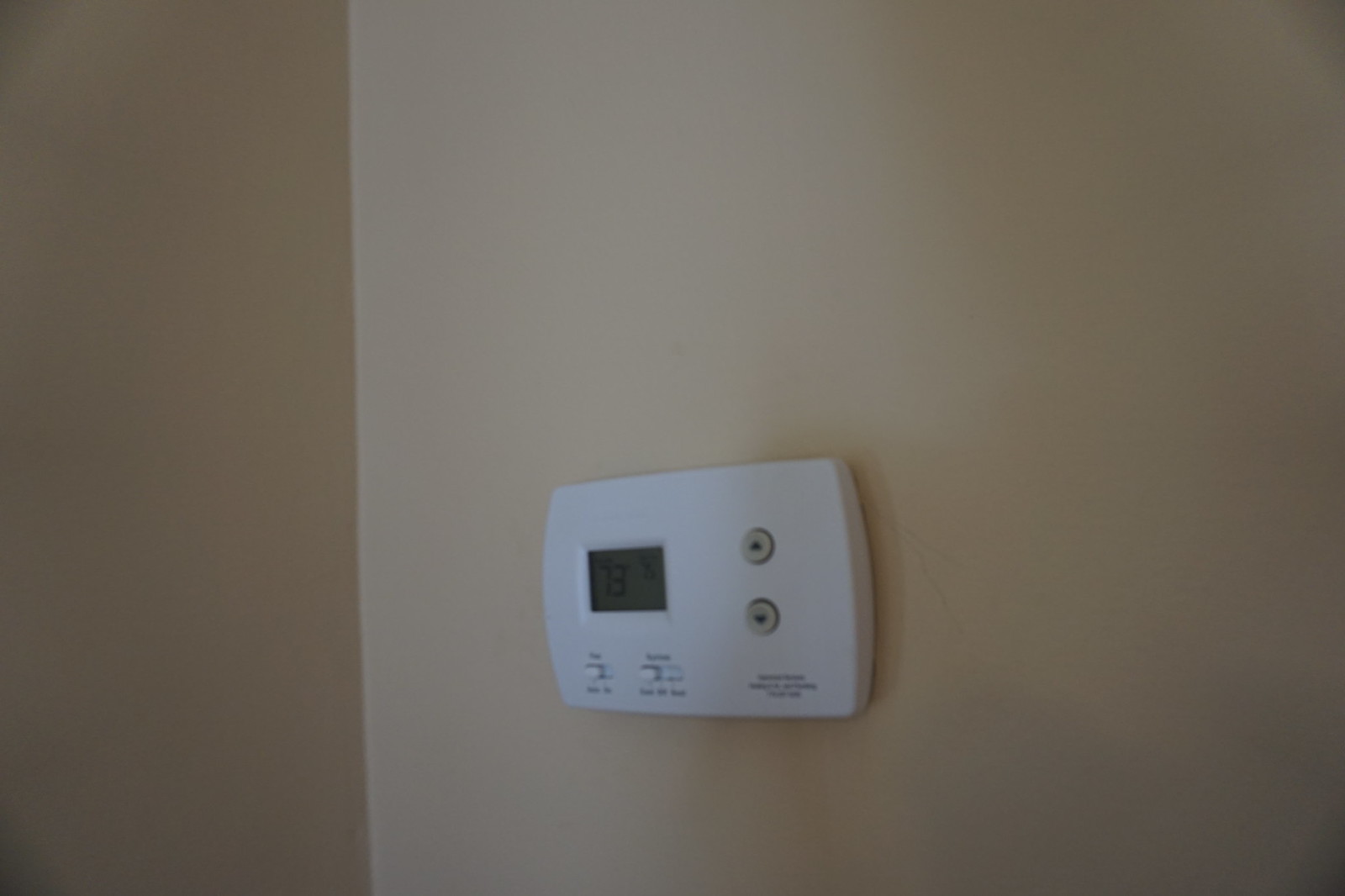The color photograph captures a seemingly mundane scene of an off-white wall corner in a landscape orientation. The wall in this corner appears to have a slightly darker tan stripe, possibly due to shadowing on the left side, while the main portion of the off-white wall occupies the remaining three-quarters of the frame. Absent of any ceiling or floor, the image focuses solely on the meeting point of the two walls, bathed in contrasting areas of light and shadow.

Dominating this unassuming composition is a white thermostat, centrally positioned within the frame on the right wall. The thermostat features a rectangular shape with slightly curved vertical edges. Prominently displayed on the left side is a digital screen indicating a temperature of 73 degrees Fahrenheit. Adjacent to the screen are two sliding switches, though their exact function is indeterminable due to their diminutive size. Completing the device, the right side showcases up and down arrows intended for adjusting the temperature setting. Below these controls, fine print details the name and contact information of the HVAC company responsible for the installation, though this text remains too small to decipher clearly.